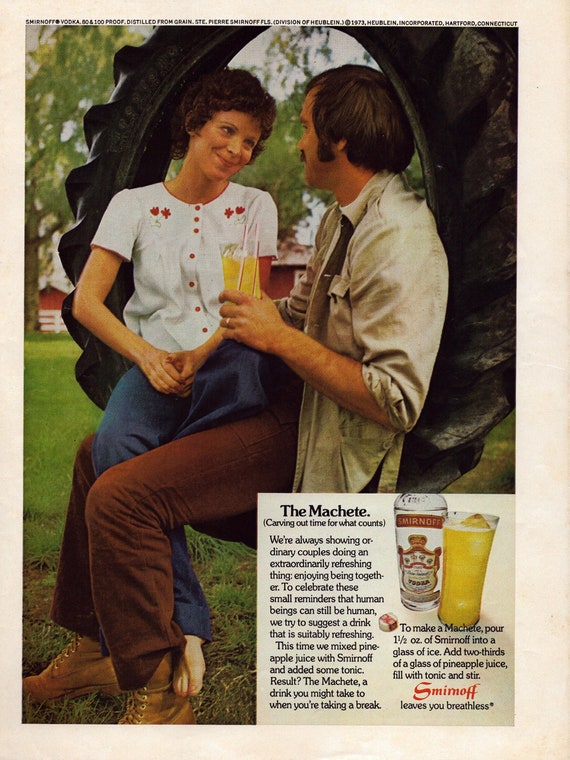This vintage Smirnoff advertisement features a full-page, sunlit photo of a loving couple sitting in a large black tire swing suspended from a tree, set against a backdrop of lush green grass and trees, with a red barn in the distance. The man, wearing brown pants, Timberland-style boots, and an open long sleeve shirt with rolled-up sleeves, is holding a glass of a Smirnoff beverage. He has short hair with long sideburns, a mustache, and a wedding ring on his left hand. The barefoot woman, with a short curly pixie cut, is dressed in a cap sleeve white top adorned with red floral appliques and buttons, paired with blue jeans. She has her legs draped across the man's lap, and they gaze lovingly into each other’s eyes. In the bottom right corner, there's a white box with the text "The Machete, carving time out for what counts," along with a recipe for the Machete drink from Smirnoff, featuring a bottle of Smirnoff and the brand's logo. The recipe instructs to pour one and a half ounces of Smirnoff into a glass of ice, add two-thirds of a glass of pineapple juice, fill with tonic, and stir. The text emphasizes that Smirnoff "leaves you breathless."